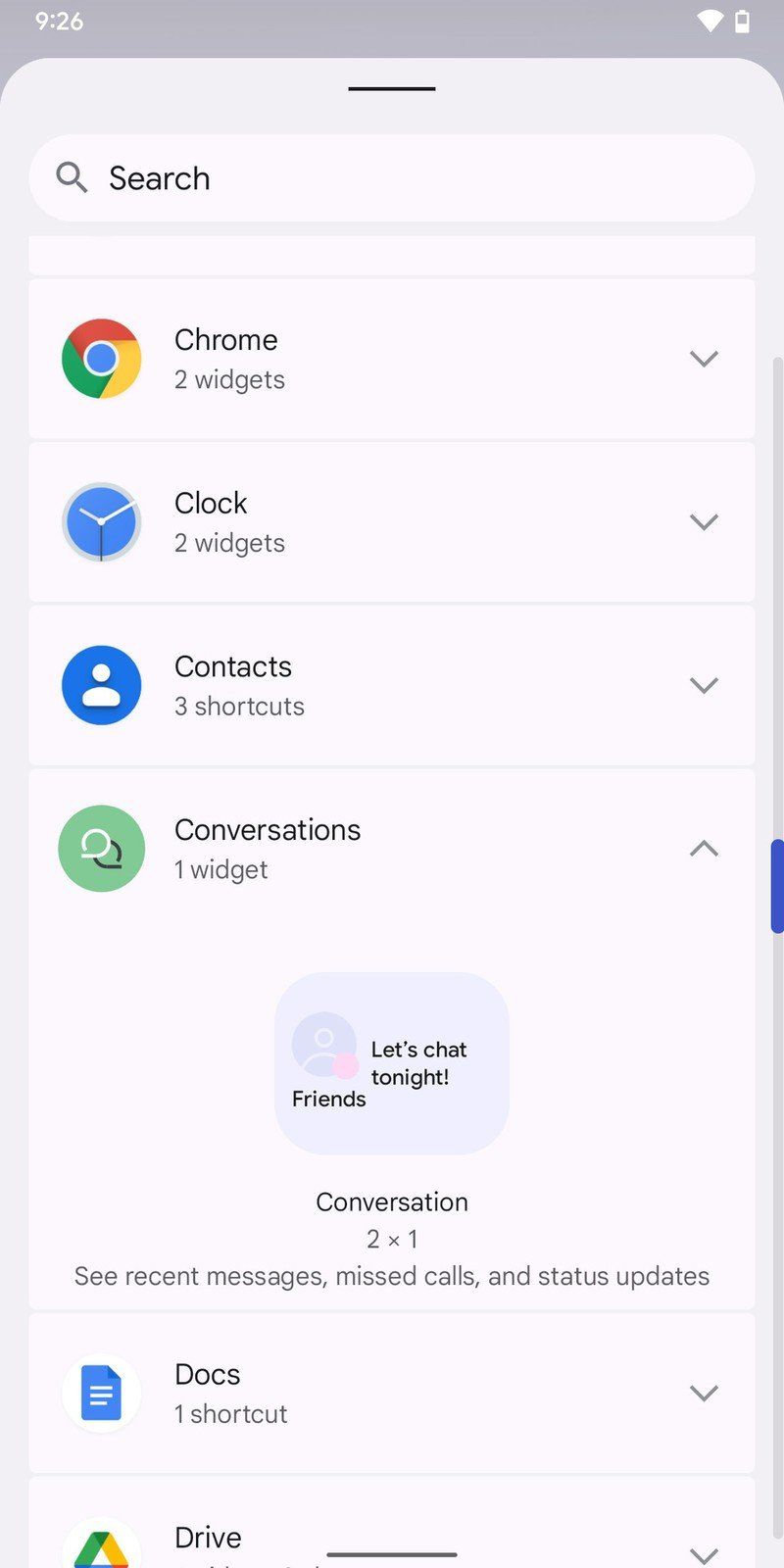Screenshot of a Google phone displaying the settings or installed apps page. At the top of the list is the Chrome app, which includes two available widgets. Following Chrome, the Clock app is listed with two widgets, and then the Contacts app with three shortcuts. The Conversations section is also visible, and its dropdown menu has been expanded. Within this dropdown, it indicates that there is one widget available. The detailed area in the center of the menu shows a widget labeled "Let's chat tonight, friends" with a size specification of 2x1. This widget displays any recent messages, missed calls, and status updates, which can be added to the home screen of the smartphone. The page overall provides various options for adding shortcuts and widgets to customize the smartphone’s home screen.